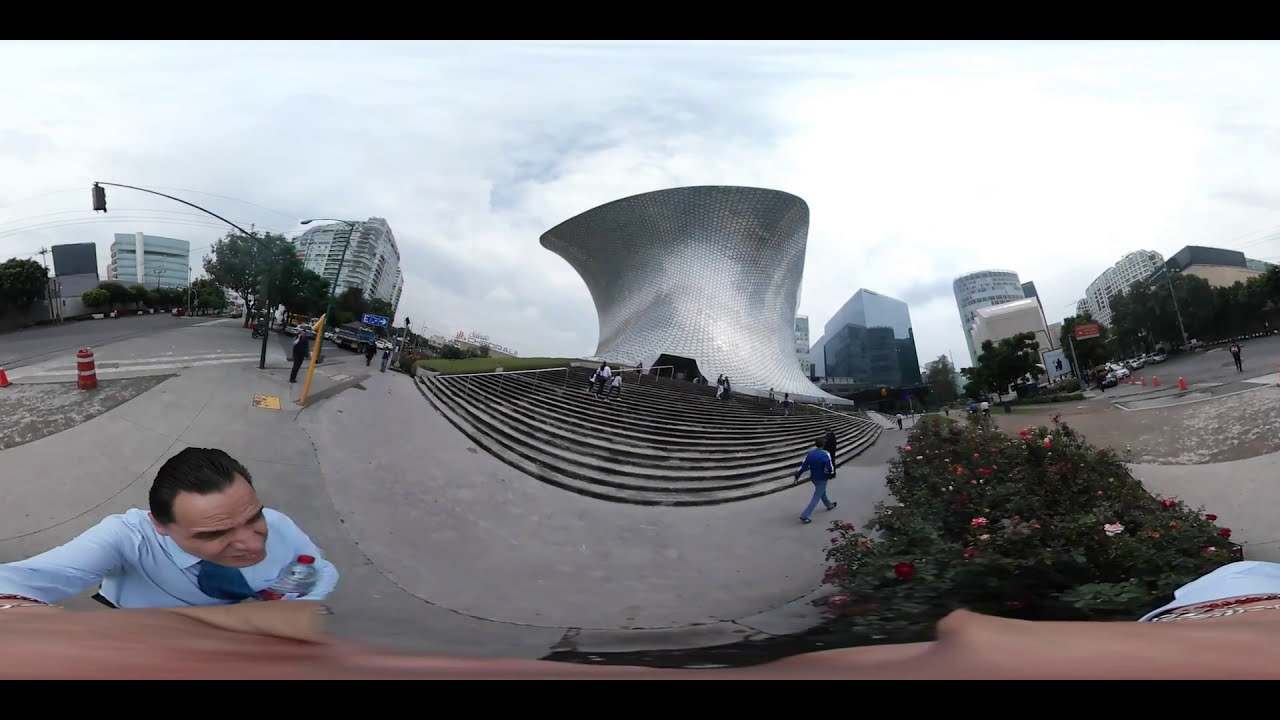This photograph captures a dynamic, urban park scene with a manipulated, possibly fisheye or panoramic view that gives a curved appearance. At its center stands a striking silver cylindrical sculpture with a unique curve in the middle, set atop approximately 25 steps. The setting is an outdoor street area with green walking paths bordered by roads bustling with vehicles. On the right side, a man in a light blue shirt, dark blue tie, and holding a water bottle—likely the photographer—appears elongated due to the image's distortion. Surrounding the park are various city buildings, including larger structures to the left and a visible stop sign. A bush with red berries adds a touch of nature in the foreground. The day is slightly overcast, with a white and blue sky dotted with clouds, creating a pleasant yet dynamic atmosphere. People are scattered around, walking and enjoying the day, enhancing the lively urban park ambiance.